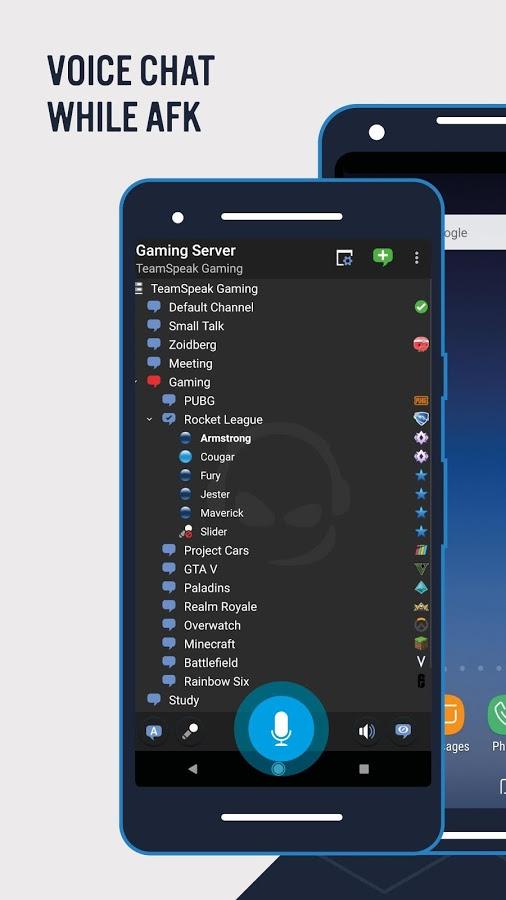Here is the cleaned-up and detailed caption for the image:

---

The image appears to be an advertisement for a mobile phone application, set against a sleek gray background. Featured prominently are two smartphones. 

The phone in the background showcases a grayish-black screen with a search bar located at the very top. At the screen's bottom, notable icons, including a phone symbol and an images symbol, are visible.

The second phone, almost entirely covering the first, provides a clearer view. A white banner at the top of this phone reads “Gaming Server, TeamSpeak Gaming” with a green plus sign positioned to the right of the text. Below the banner, multiple folder options are neatly displayed. The list includes "TeamSpeak Gaming" followed by a variety of channels:

1. **Default Channel**
2. **Smalltalk**
3. **Zoidberg**
4. **Meeting**
5. **Gaming**:
   - PUBG
   - Rocket League
     - Armstrong
     - Cougar
     - Fury
     - Jester
     - Maverick
     - Slider

Further down, additional folders are displayed:

6. **Project Care**
7. **GTAV**
8. **Paladine**
9. **Realm Royale**
10. **Overwatch**
11. **Minecraft**
12. **Battlefield**
13. **Rainbow Six**
14. **Study**

At the bottom of the screen, there is a blue circular icon featuring a microphone, likely indicating the voice chat functionality. Text in the upper left corner of the image highlights the feature “Voice Chat While AFK.”